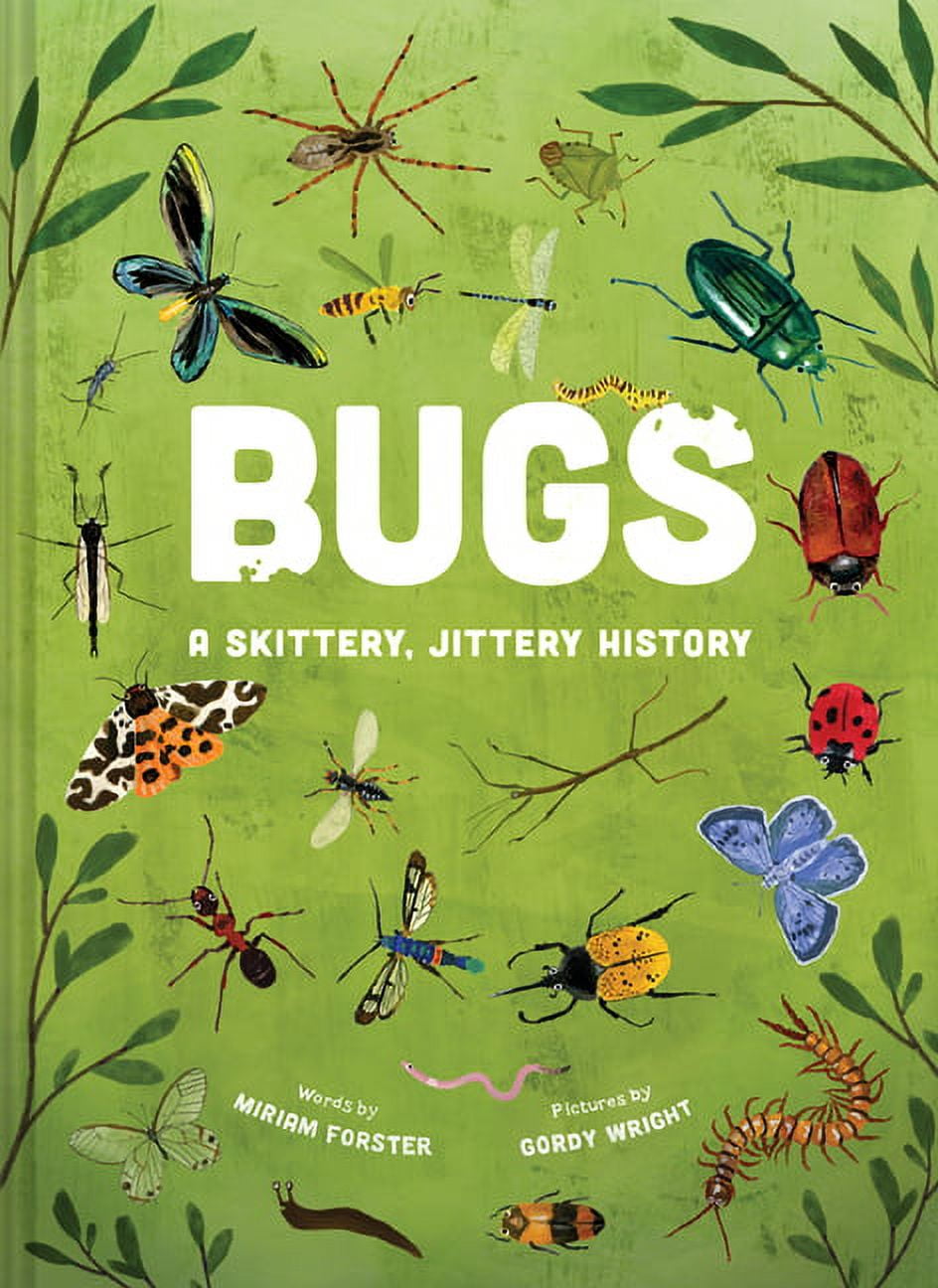The cover of the children's book "Bugs: A Skittery Jittery History" is an artistic, nature-themed design featuring a light green background adorned with branches and leaves. Dominating the center of the cover is the title in large white letters. Along the bottom, in white text, it reads "words by Miriam Forster" on the bottom left and "pictures by Gordy Wright" on the right. The cover is lively with vivid illustrations of various insects. In the top left corner, there is a large green and yellow butterfly. To the right, there are three distinct beetles and a red ladybug with black spots near the middle right. A sandy peach-colored insect is located in the bottom right. In total, there are 18 detailed bug illustrations, bringing splashes of color with greens, whites, blacks, reds, blues, and yellows, making this book cover highly engaging for young readers.